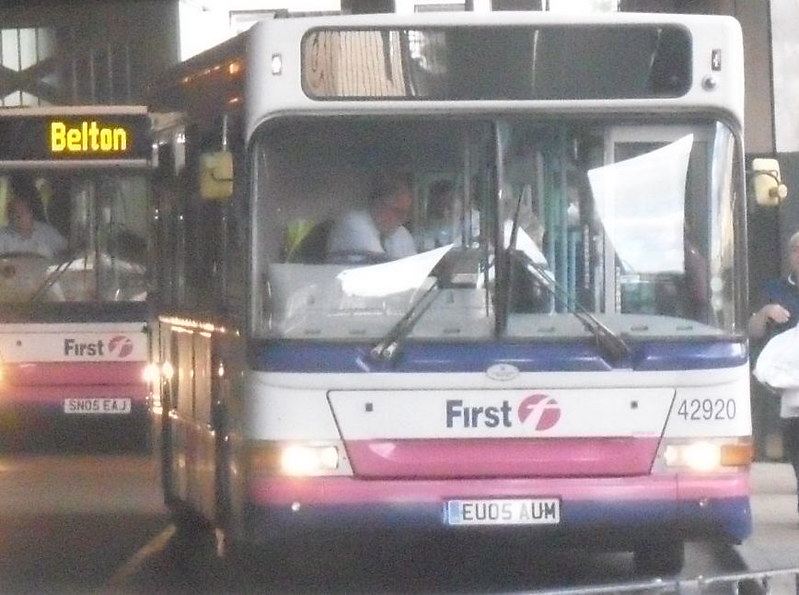The photograph depicts a somewhat poorly lit and slightly out-of-focus, full-color scene that takes place outdoors during the daytime, likely in Europe, specifically England. The image, which is horizontally rectangular with no border, captures two white buses with a blue stripe in the middle and a white stripe just beneath the large windows, each equipped with prominent windshield wipers. Both buses belong to the "First" brand, denoted by the name on their fronts, accompanied by a red circle with a cross through it.

In the foreground, there is an older white male bus driver, positioned on the left side of the bus, consistent with European driving norms. He is looking down, and the electronic display on his bus is not illuminated to show any destination. This bus features a European-style license plate, specifically reading "EUDS5AUM," and it is numbered 42920.

Behind the front bus, a second identical bus is visible. Its electronic sign is lit up with the destination "Belton," indicating the bus’s route. Another older male driver wearing glasses is seen behind the wheel of this bus. The bus doors are closed, suggesting that the scene captures a moment when no passengers are boarding. Additionally, a person holding a bag is visible in the background, seemingly waiting to get on one of the buses. The overall setting appears to be a bus station in England, with the buses driving on what would be considered the left side of the road in Europe.